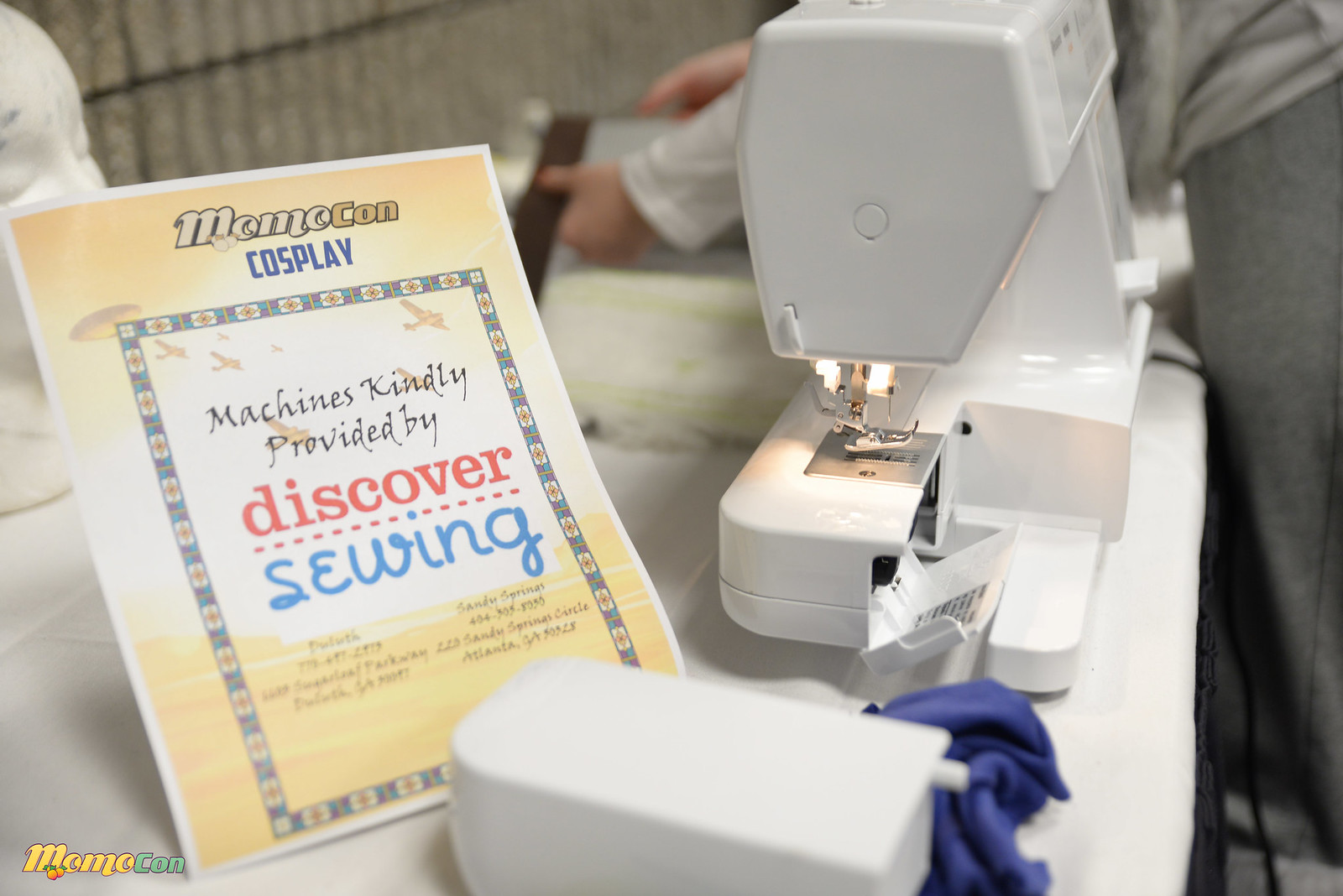The image features a modern, white sewing machine situated on the right side against a white table, appearing almost brand-new with a light illuminating the stitching area. The machine is partially open, revealing a shiny plastic exterior and an open compartment. To the left of the machine, a beige and white sign reads "Momocon Cosplay. Machines kindly provided by Discover Sewing" in black text, with further contact information at the bottom. The sign leans against a white mannequin head positioned towards the table's rear. In the background, a person dressed in gray sweats and a gray shirt is visible, handling a piece of white fabric, possibly folding a dress. The upper left corner of the image shows a gray stone wall. Additionally, there's a book with a yellow and white background featuring the red title "Discover" and the blue subtitle "Sewing," surrounded by a blue and red border, with "memo.com" written at the bottom. The scene captures a detailed and organized sewing workspace with various elements contributing to a focused crafting atmosphere.